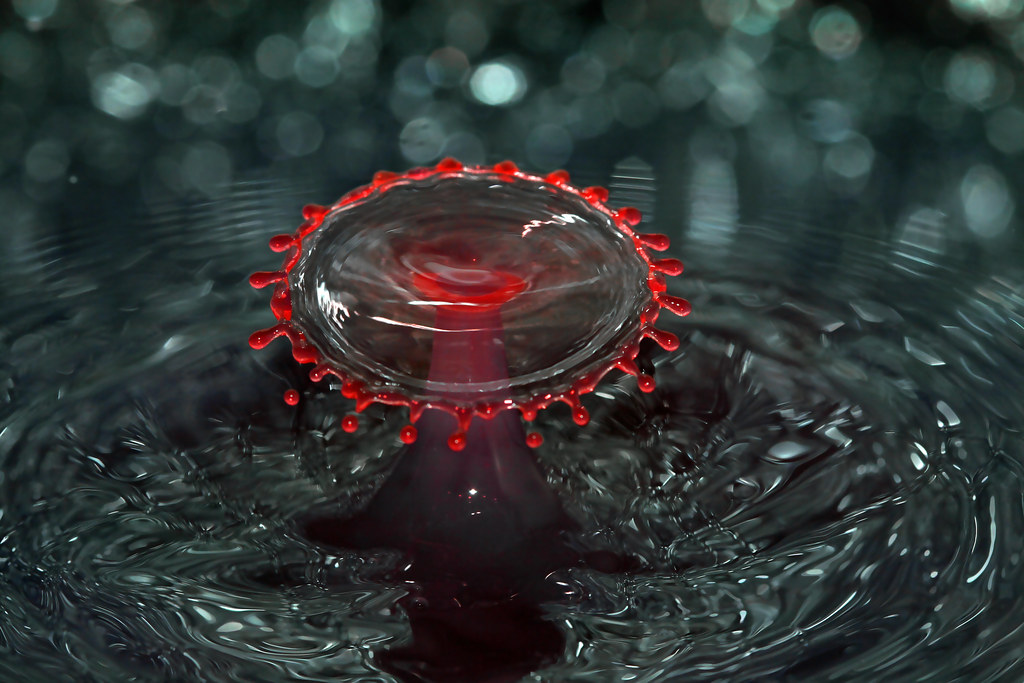In this highly detailed and dynamic photograph, we're observing the instant when an object has just been dropped into a pool of water, capturing the vivid interaction between the drop and the water's surface. Central to the image is the dramatic impact zone, characterized by a deep divot where the object broke the surface, creating a focused area of disturbance. From the center of this divot, a striking upspurt, reminiscent of an upside-down cone or a pedestal, rises prominently. This upspurt features a bright red hue at its peak, which subtly diminishes into darker shades as it cascades down into the surrounding water.

Encircling the upspurt is a series of concentric rings, akin to those formed when skipping a rock across the water, spreading outward and illustrating the ripple effect of the splash. The fluid in the impact area appears cohesive, with smooth, still water seemingly connecting inside the inner circle.

Adding to the visual spectacle are droplets, also a vivid red, that can be seen flying off the edge of the upspurt. These droplets, caught in mid-air, hint at their impending return to the surface of the water. The combination of colors and motion captured in this moment creates a stunning interplay of light and water, emphasizing the natural and fleeting beauty of the scene.